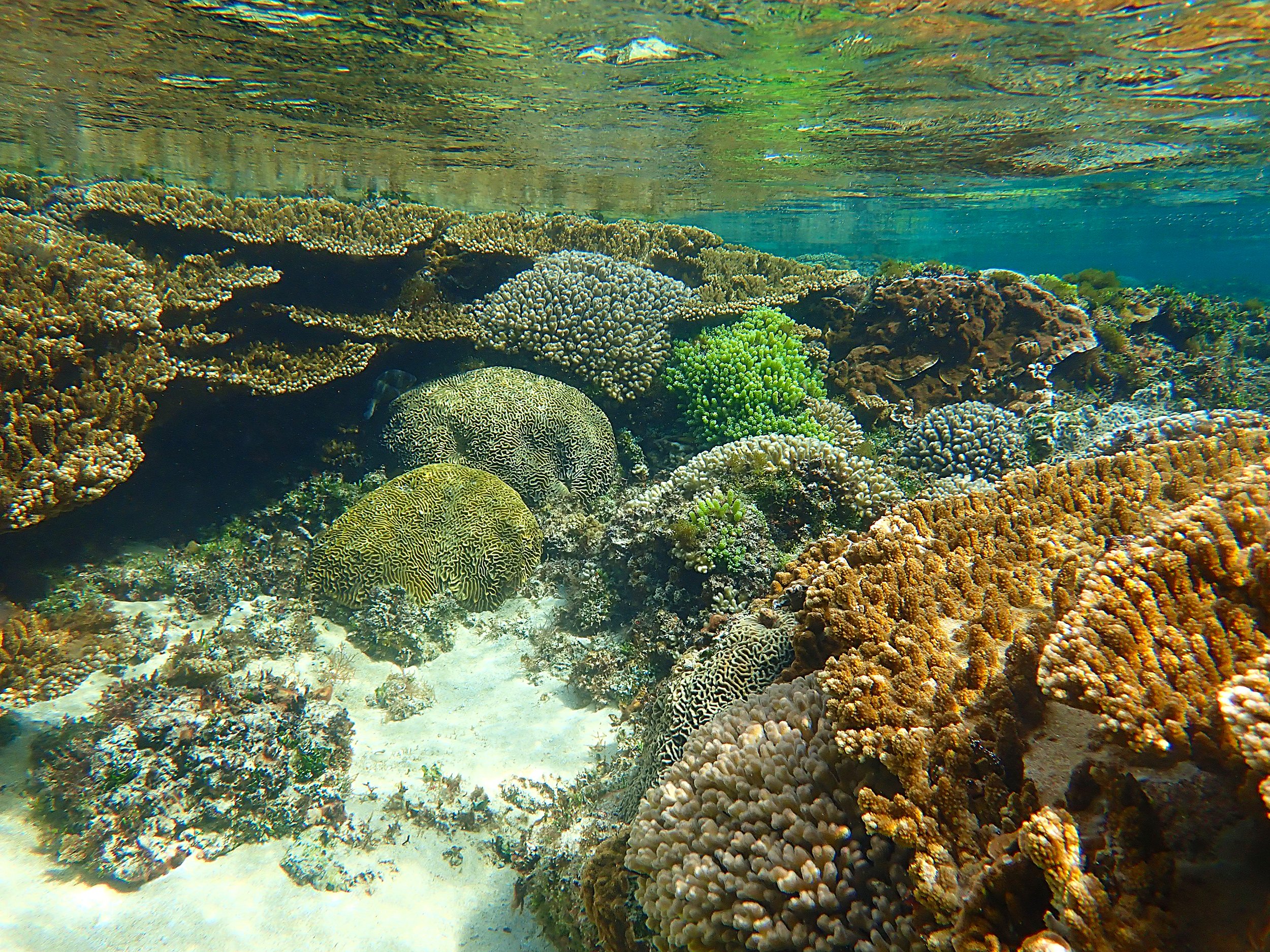An underwater image reveals an intricate scene teeming with vibrant coral and sea vegetation. Predominantly showcasing a variety of corals, the shot spans the ocean floor, displaying hues of green, brown, orange, and dark green, flecked with lighter shades. The coral formations and plants extend from left to right, occasionally interrupted by sandy patches and rocky outcrops covered in algae. The water above is exceptionally clear, allowing visibility of a mirrored reflection of the underwater life on its surface. Amidst the calm, blue-green water, no fish are present, leaving the focus solely on the colorful sea floor. Adding a unique touch to the scene, a sprinkling of snow is visible on part of the image, hinting at a wintry landscape above the water, which contrasts with the lush underwater greens and the clarity of the ocean.